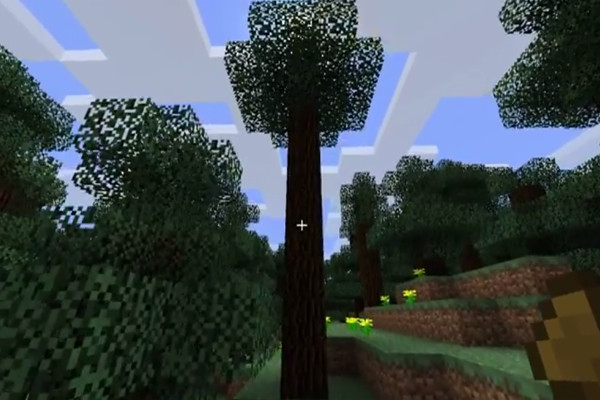The image is a screenshot from a three-dimensional video game, likely Minecraft or Roblox. The scene features a lush forest with numerous trees, their leaves forming a dense canopy. Nestled within the forest is a tiered garden bed, meticulously structured on different levels, each adorned with vibrant yellow flowers. The sky overhead is a clear blue, populated with geometric clouds in rectangular and square shapes, adding to the game's blocky aesthetic. At the very center of the image, a small white cross serves as a focal point, perhaps indicating a cursor or a point of interest within the game. The bottom right corner subtly includes the indistinct hand of a character, though it remains nondescript and does not draw attention away from the detailed environment. The image lacks any textual elements, allowing the intricate and colorful visuals of the virtual world to speak for themselves.